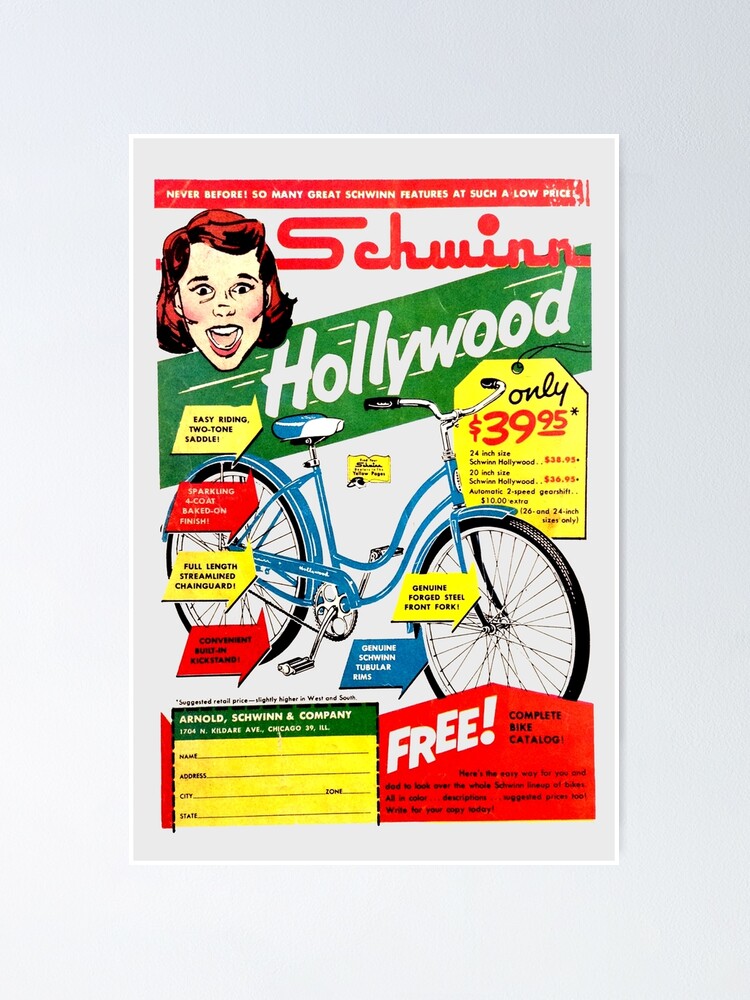This advertisement for the Schwinn Hollywood Bicycle is a vibrant, detailed flyer showcasing a vintage design with vivid colors—reds, whites, greens, blues, and yellows. At the very top, the banner proclaims, "Never before so many great Schwinn features at such a low price." The upper left corner features an illustration of a young woman with very red hair, her mouth open in excitement. Below, in a red cursive font, the Schwinn name appears prominently, followed by "Hollywood" on a green, slanted banner running from left to right.

The centerpiece of the ad is the Schwinn Hollywood Bicycle itself, depicted in blue with a blue and white seat, and black handlebar grips. Emphasizing affordability, the ad states, "Only $39.95, 24-inch size Schwinn Hollywood," though a few specifics on smaller 20-inch models are unclear. Red and yellow arrows point to key features such as the "easy riding two-tone saddle," "sparkling four-coat baked-on finish," "full-length streamlined chain guard," "convenient built-in kickstand," and "genuine forged steel front fork."

The bottom section of the ad includes a cutout mail-in form for potential buyers to send to Arnold, Schwinn, and Company at their address, "1704 North Kildare Avenue." The form asks for personal details like name, address, city, state, and zip code. In the bottom right corner, a red house-shaped box with a rooftop design highlights a promotional offer with the words, "Free complete bike catalog," providing further ordering details. The entire flyer is bordered by a thick light gray frame, enhancing its antique, collectible appearance.